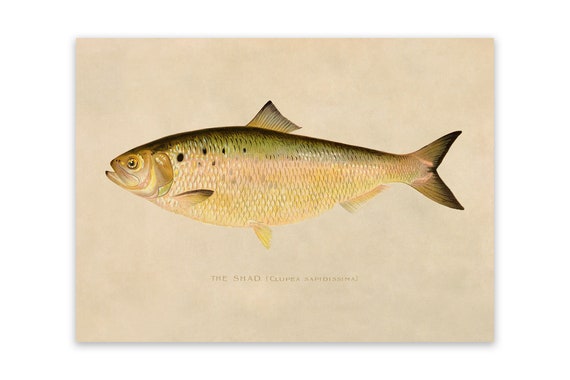This image is a detailed illustration of a fish known as "the shad" (Clupea sapidissima), depicted against a light pink background with a paper-like texture. The fish has a gradient coloration, with a green back that fades to a yellowish white belly. Its body features a distinctive black stripe running from head to tail, and there are several spots near its head. The fins include a green dorsal fin, yellow pectoral fins, and a tail that transitions from light brown to black at the tips. The fish has small fins close to its head and two additional fins near the back. Its tail and top fin are outlined in black. Notably, the fish's eyes are yellow and its mouth is open, facing the left side of the image. Below the fish, in green lettering, is the text "the shad" followed by its scientific name in parentheses: "Clupea sapidissima."